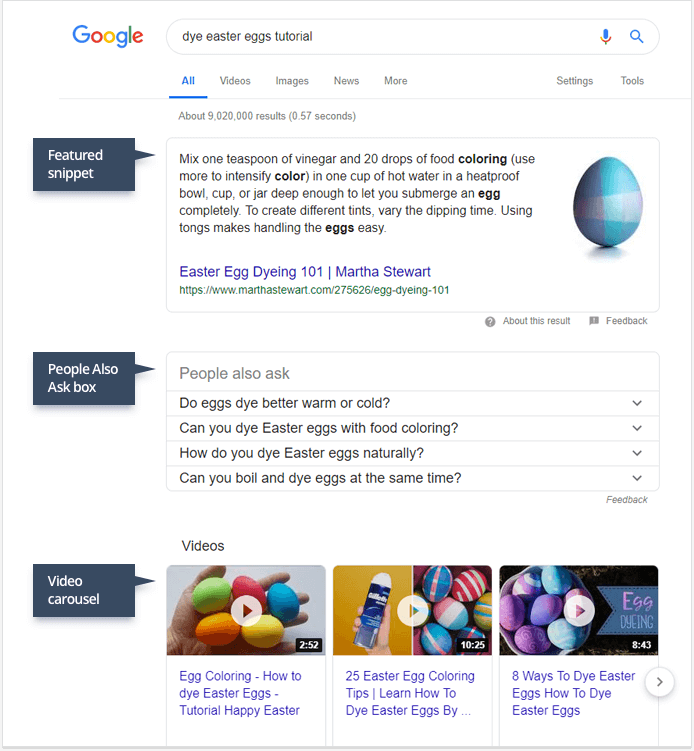The image depicts a screenshot of a Google search related to Easter egg dyeing tutorials. The background is completely white, with the iconic multicolored Google logo displayed in the upper-left corner. The search query entered is "Die Easter Eggs Tutorial."

Beneath the search box, there are several tabs: "All" (highlighted in blue, indicating the current active tab), followed by "Videos," "Images," "News," "More," "Settings," and "Tools" in gray.

The search results return approximately 9,020,000 results in 0.5 seconds. The left section features a "Featured Snippet" outlined in light gray. This snippet contains instructions on dyeing Easter eggs: "Mix 1 teaspoon of vinegar and 20 drops of food coloring (use more to intensify color) in one cup of hot water in a heatproof bowl, cup, or jar, deep enough to submerge an egg completely. To create different tints, vary the dipping time. Using tongs makes handling the eggs easy." Below these instructions, the snippet attributes the source to "Easter Egg Dying 101" from Martha Stewart, clickable in blue, with a hyperlink to the Martha Stewart website.

On the right side of the Featured Snippet, there's an image of a light blue egg, and below it, the text "About this result" and "Feedback."

Further down, a dark gray "People also ask" box with white text displays common related questions, which can be expanded: 
- "Do eggs die better warm or cold?"
- "Can you dye Easter eggs with food coloring?"
- "How do you dye Easter eggs naturally?"
- "Can you boil and dye Easter eggs at the same time?"

Beneath this section, to the right, there's another "Feedback" option.

Moving further down, the next section is a video carousel with a dark gray background and the heading "Videos" in white. It features three horizontally-aligned videos, each with a play symbol:

1. The first video shows a person holding five dyed Easter eggs (green, reddish-pink, blue, orange, and yellow). The video is titled "Egg Coloring. How to Dye Easter Eggs Tutorial Happy Easter" and lasts 2 minutes and 52 seconds. It's clickable via a blue hyperlink.
   
2. The second video, 10 minutes and 25 seconds long, shows someone holding a can of Gillette shaving cream and various dyed Easter eggs. It is labeled "25 Easter Egg Coloring Tips. Learn How to Tie Easter Eggs By" and is also clickable in blue.
   
3. The third video features a bowl of pastel-colored Easter eggs (purple and light blue). It's 8 minutes and 43 seconds long and titled "8 Ways to Dye Easter Eggs. How to Dye Easter Eggs," also hyperlinked in blue.

The screenshot, overall, indicates that the user is searching for comprehensive tutorials on how to dye Easter eggs for the Easter celebration.